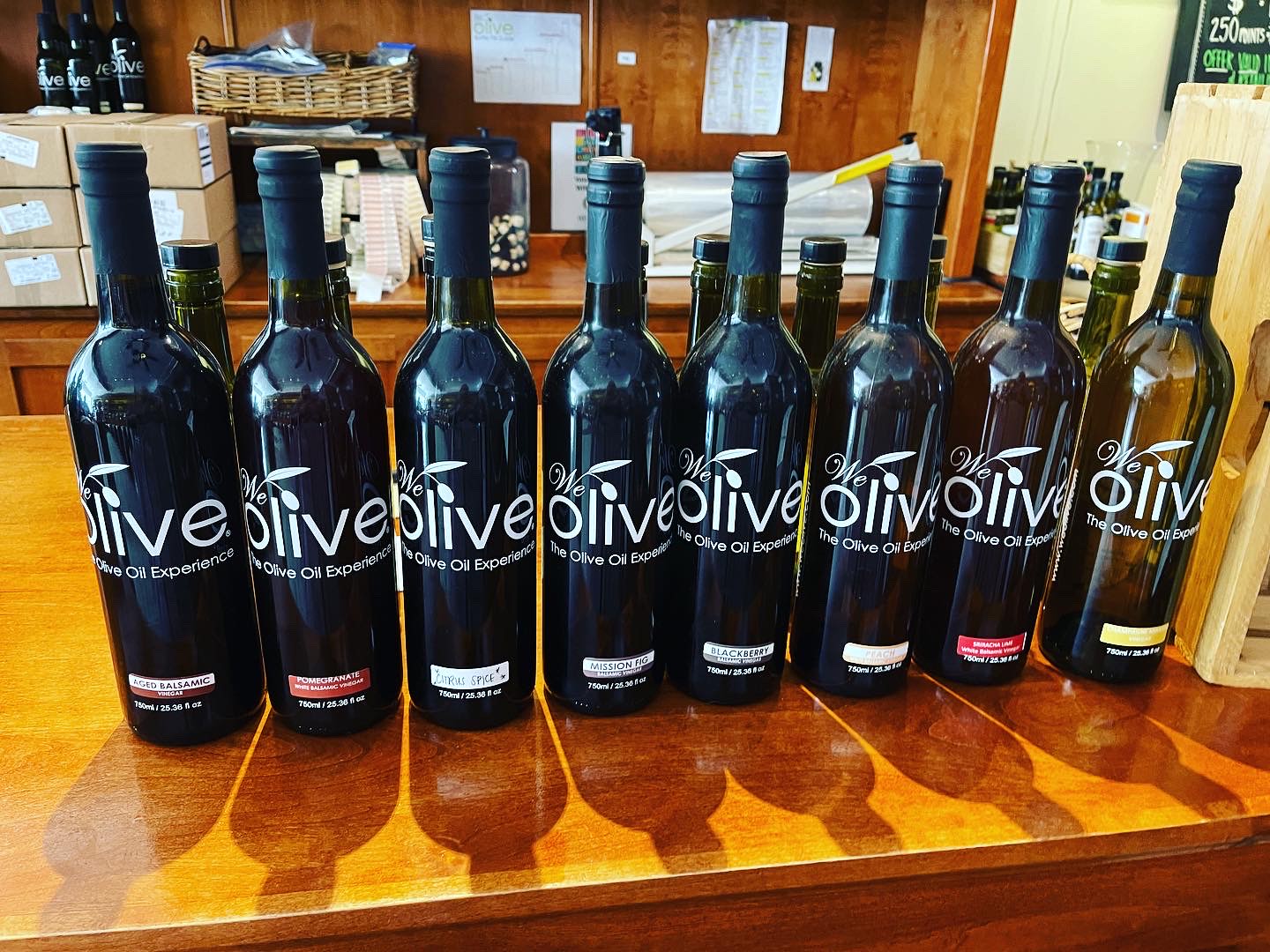This color photograph captures a display of eight olive oil bottles arranged in a row on a wooden table. The table features a shiny light brown top and a darker brown front, visible at the bottom of the image. The seven bottles on the left are dark blue, while the eighth one on the far right is slightly transparent with hints of blue and orange. Each bottle displays the label "We Olive" in white lettering, with "Olive Oil Experience" written beneath in smaller font. A varying label at the bottom of each bottle denotes the different flavors, including Aged Balsamic Vinegar, Pomegranate Balsamic Vinegar, Citrus Spice, Mission Fig Balsamic Vinegar, Blackberry Balsamic Vinegar, Peach, and Sriracha Lime White Balsamic Vinegar. The last label is indistinct but yellow with white writing. Behind the row of bottles, the necks and black caps of smaller green-necked bottles are visible, along with a shelf that holds various boxes and papers taped to the wall. The shelf itself is a dark brown wood, adding depth to the background.